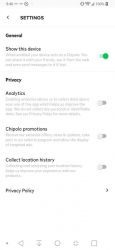A blurry screen capture displays a settings page on a mobile device. At the top, the word "Settings" appears in black, accompanied by a black arrow pointing left, indicating a return option to the home page. The background is white, and the top status bar shows indistinct icons for internet connectivity, cellular signal, battery level, and the time.

The screen lists various menu items starting with “General,” followed by a section that likely reads "Show This Device," accompanied by a green toggle switch indicating it is enabled. Below that, there is the word "Privacy," leading into another section titled "Analytics," with a toggle switch set to on, and accompanying blurred gray text.

Further down, there seems to be a mention of "Chipotle Promotions," though this is unclear, with another toggle button to the right. Next is "Collect [Something] History," with additional illegible text and a toggle button that is in the off position.

At the bottom of the screen, "Privacy Policy" is listed with a clickable arrow for more information. The very bottom features icons that represent volume, the home button, and other functions, though these are also difficult to discern due to the blurriness.